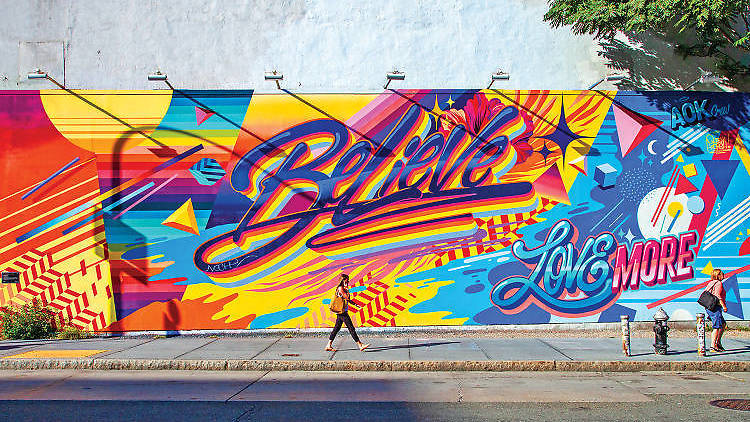The image portrays a vibrant urban street scene featuring a colossal, brightly painted mural along a city sidewalk. The mural, adorned with dynamic shades of orange, yellow, blue, and red, prominently displays the words "Believe" and "Love More." The word "Believe" is particularly striking, with blue letters accompanied by a rainbow gradient, while "Love More" is stylishly divided, with "Love" in blue and "More" in red. Above the mural, seven lights are lined up, casting illumination over the painting, which extends across a vast expanse of the wall. 

Walking along the sidewalk in front of the mural are two women. One woman, carrying a black purse, appears to be engaged with her cell phone. The other, slightly ahead and to the right, is carrying a brown purse and gazes upward, seemingly captivated by something in the sky or the surroundings. Further details in the scene include a fire hydrant and two posts situated on the right side of the image. The upper right corner of the photograph shows a portion of tree branches and leaves, adding a touch of nature to the urban setting.

The mural, with its immense size and vibrant color palette, appears far larger than typical billboards, capturing the attention of passersby and adding a lively artistic element to the street.